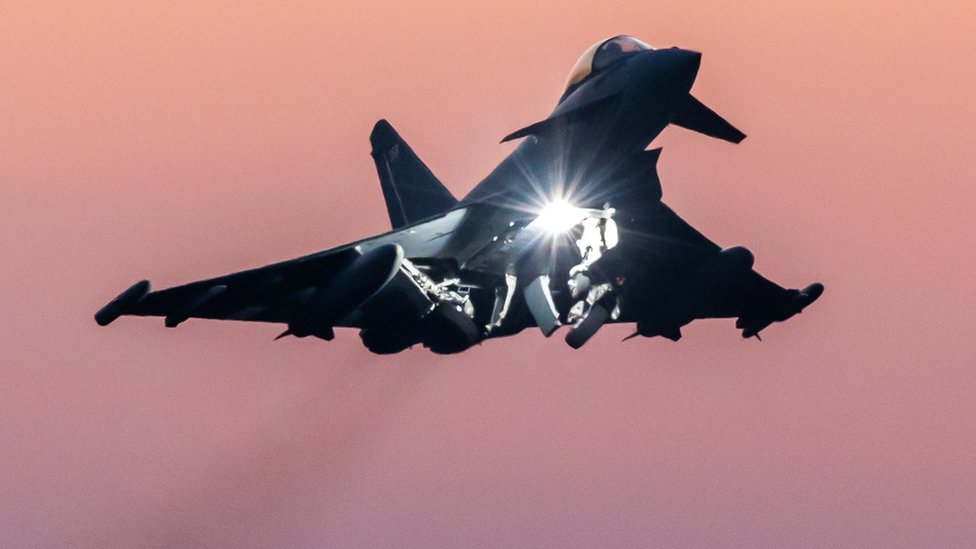This photo captures the dramatic underside of a dark aircraft in flight, possibly resembling a fast jet or military plane, with partially deployed landing wheels and flaps. The setting sun paints the sky in a spectrum of warm hues, transitioning from a peachy rose in the top left to a deeper burgundy pink in the bottom right. A bright landing light shines from the center underneath the aircraft, casting a small, distinct glow on the cockpit glass and parts of the underbelly, which are otherwise cloaked in shadow. The overall impression is one of a silhouette against the colorful dusk sky, emphasizing the stark contrast and dynamic details of the scene.